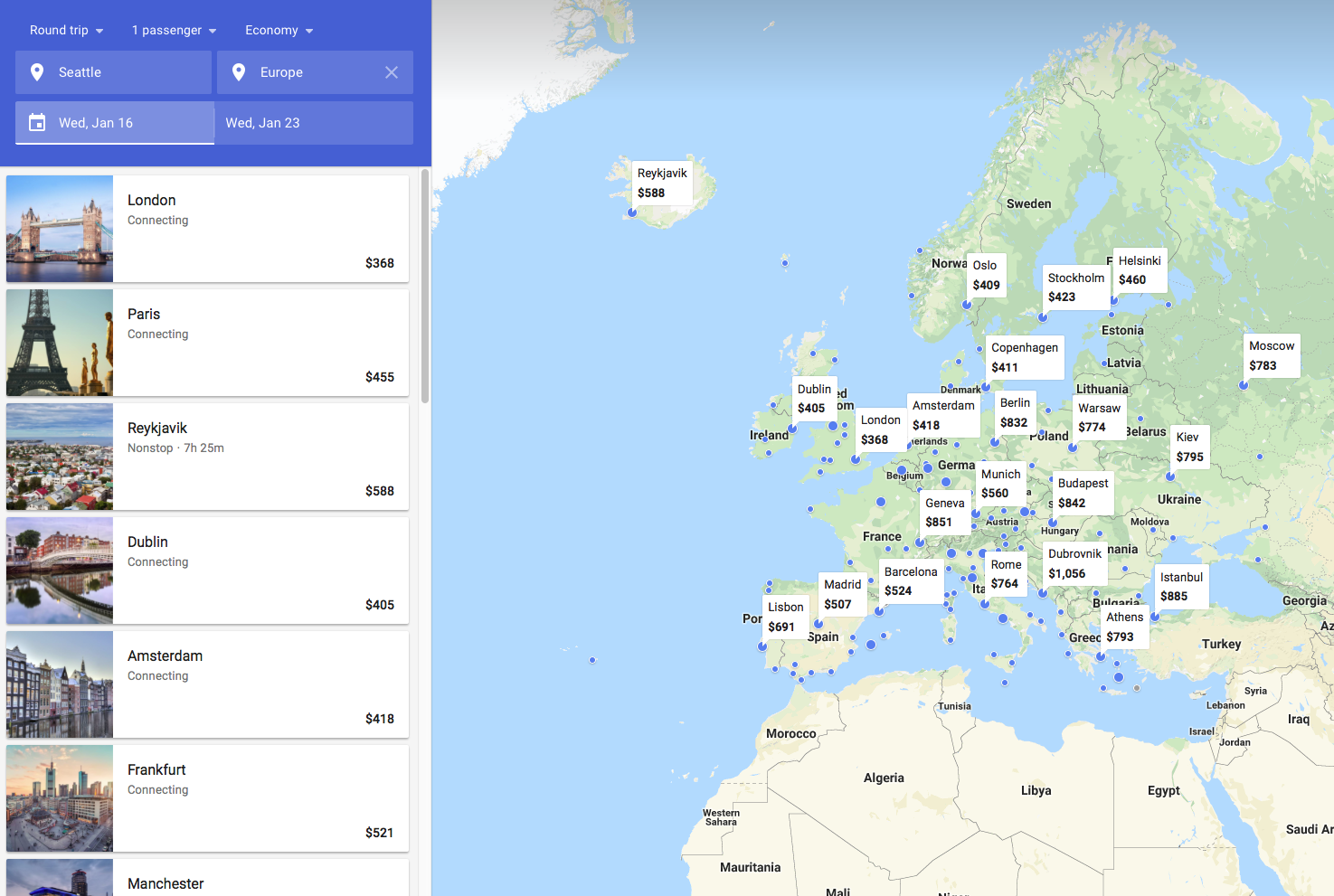The image is a horizontal rectangular screenshot from a travel website. On the right-hand side, occupying about two-thirds of the frame, is a detailed map showcasing various European destinations with corresponding flight prices. The outermost destinations and their prices include Lisbon ($691), Moscow ($783), Istanbul ($885), and Oulu ($409).

On the left-hand side, vertically, there's a list of these locations. At the top, within a prominent blue banner, are several trip customization options: trip type (round trip or one-way), number of passengers, and seating class, with economy class selected. The departure city is set as Seattle, and the destination is Europe, with the travel dates specified as departing on Wednesday, January 16th, and returning on Wednesday, January 23rd.

Below these options, there is a list of various European cities, each accompanied by a corresponding image on the left, and followed by the type of flight and its price. The listed destinations include London, Paris, Reykjavik, Dublin, Amsterdam, Frankfurt, and Manchester.